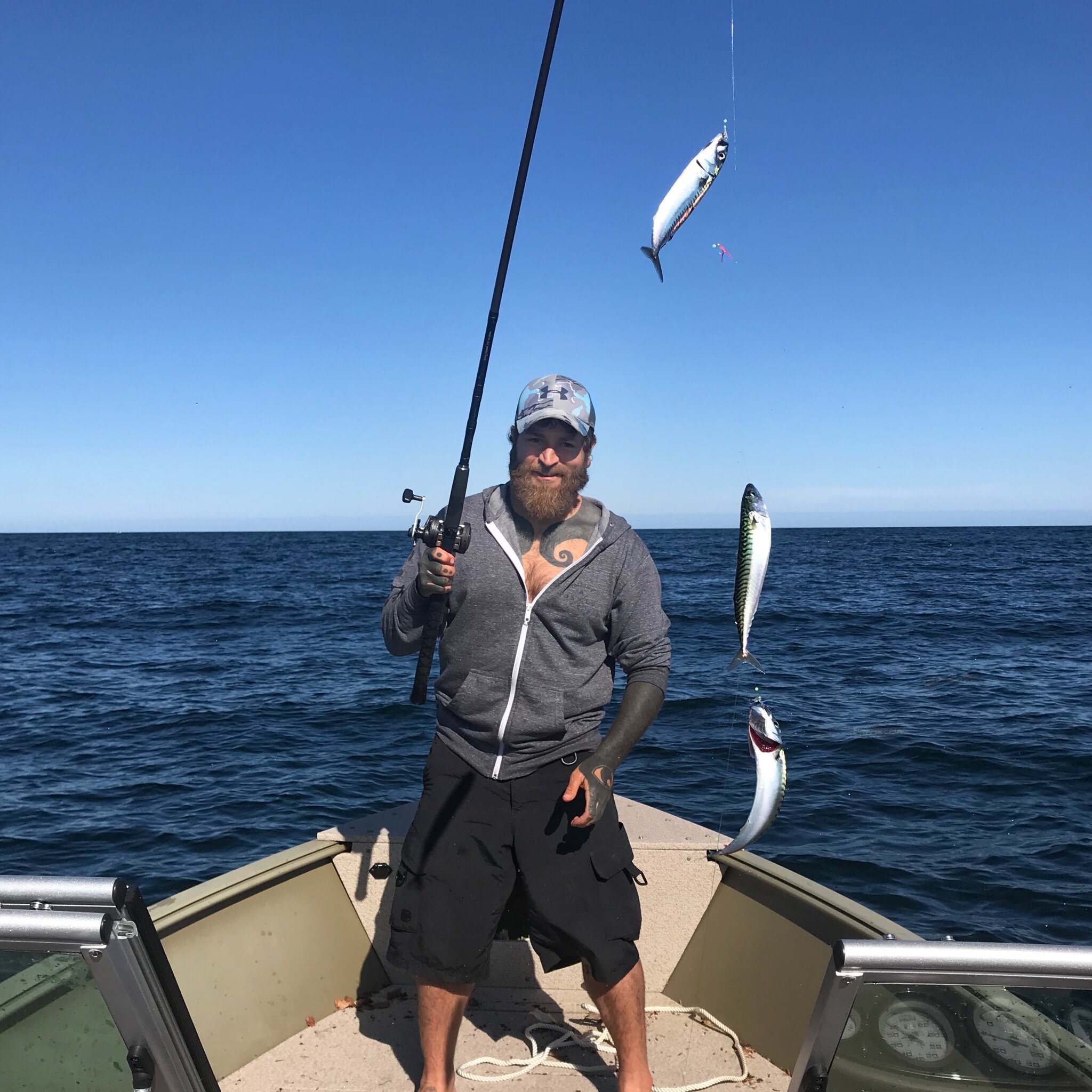In this photorealistic image, a bearded white man with a long beard and mustache is posing happily on a small fishing boat that appears to be around two or three feet wide, with tan and green hues accented with silver. He is holding a fishing rod in his right hand, which has three mid-sized silver and black fish hanging from it, indicating a successful catch. The man is dressed in black cargo shorts, a gray zip-up hoodie worn without a shirt underneath, revealing a swirl tattoo on his chest. His left arm is adorned with a full blackout sleeve tattoo that extends to part of his hand, and he has another distinctive tattoo that wraps around his neck. A silver baseball hat tops off his look. The background features a deep, vibrant blue ocean meeting an equally blue sky on a sunny day, creating a picturesque and serene setting for this fishing adventure. The man’s left hand appears immobile, giving a sense of triumph and perseverance as he stands at the hull of the boat, content with his day's catch.